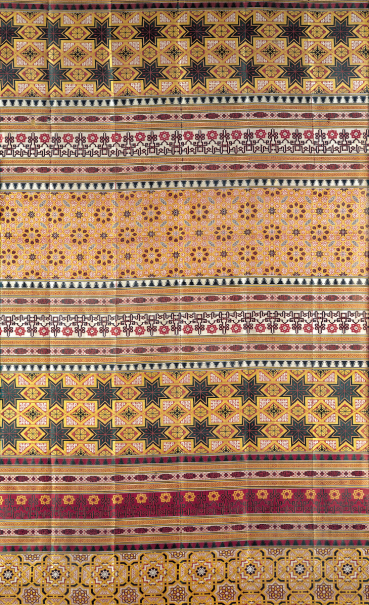The image depicts an intricate, multi-colored quilt dominated by fall shades such as dark green, yellow, red, white, tan, orange, burgundy, and various browns. The top section features a row of star-shaped patterns with black centers and yellow frames. This is followed by a thin horizontal panel decorated with smaller stars and shapes. Below that, a distinct white border with black triangles separates the next section, which consists of floral designs in reds, whites, and purples. Further down, there are panels showcasing orangish, yellowish flowers, followed by more flowers in red and yellow hues. The quilt culminates at the bottom with larger framed floral designs in yellow and black. The quilt's arrangement includes various colors and shapes creating a detailed and visually stimulating piece, evoking a sense of heritage and craftsmanship.